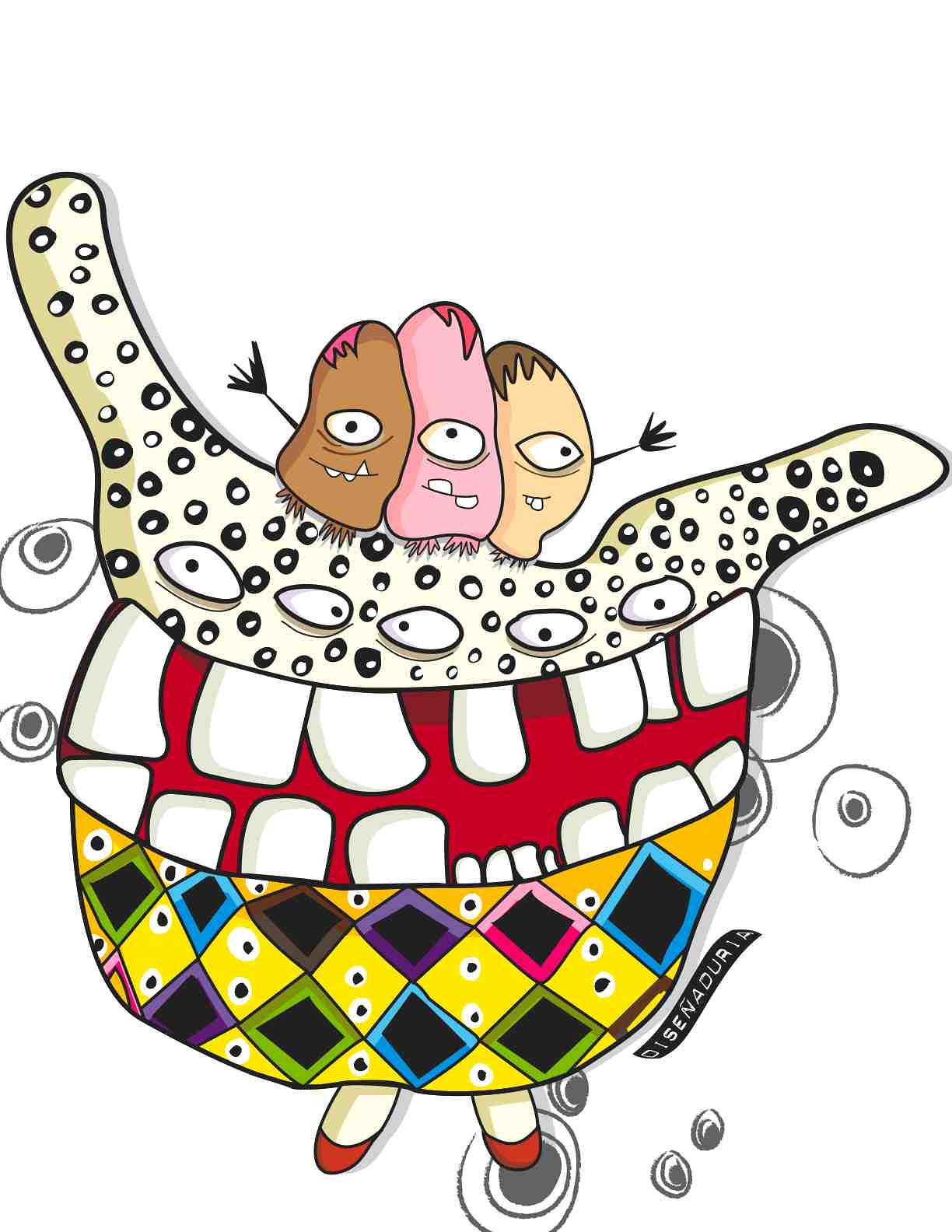The image is a colorful and detailed cartoon illustration of a fantastical beast in a square format. The character boasts a striking design with three multicolored heads, each adorned with a single eye in the center and variously colored hair—black with pink, pink with red, and white with brown—along with jutting teeth. The top half of the character's body features a red mouth partially open with white teeth and arm-like extensions in a cream color with a pattern of black and white circles. Below that is a large, rounded body resembling a belly, decorated with a diamond pattern in various colors such as yellow, green, brown, purple, pink, and turquoise blue, along with eye-like motifs. The character wears a skirt that prominently displays the yellow color amidst a mosaic of broken tiles of different hues. Its small red shoes peek out from beneath. Surrounding the figure are random circles in gray and white. An inscription reading "DICENADURIA" is placed beside the figurine, accentuating the fantasy style of the illustration.